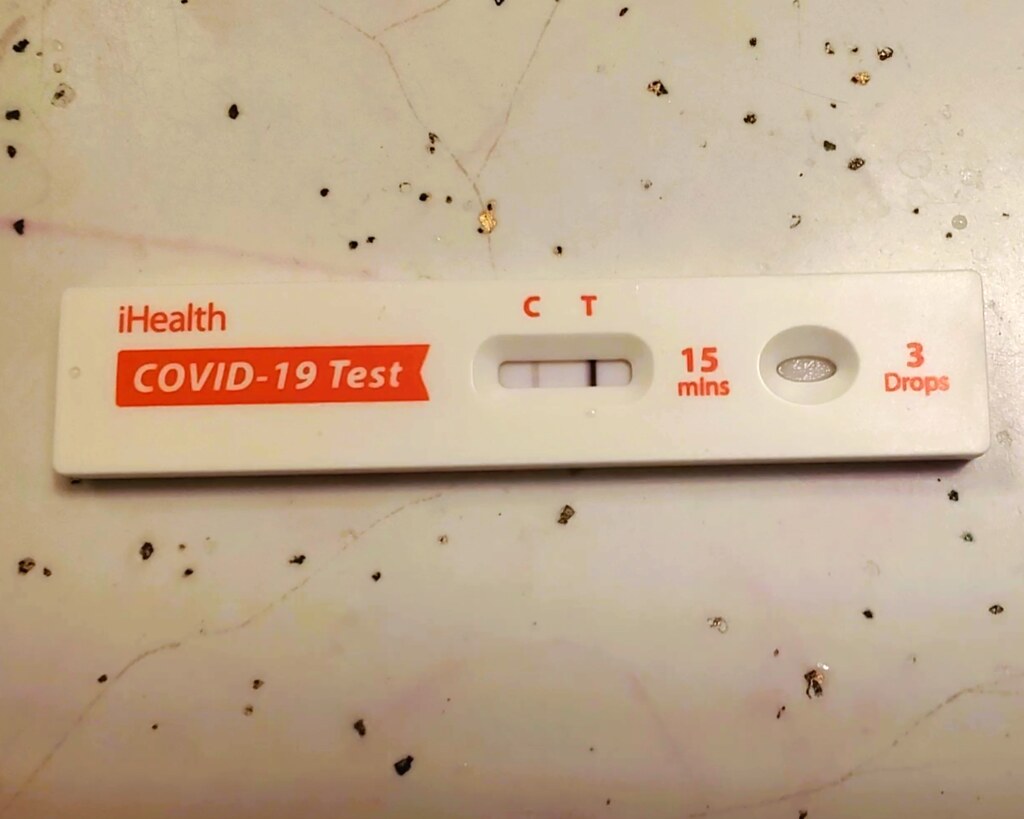This overhead photograph showcases a COVID-19 testing strip placed on a slightly textured, marbled countertop adorned with black and gold flecks. The testing strip, a small rectangular device, features the brand name "iHealth" in red text with a lowercase 'i' and an uppercase 'H' at the top left corner. Directly beneath this branding, there is a red background with "COVID-19 Test" prominently displayed in white text. 

Central to the test strip is the result window, which shows one faint line and one darker line, with the labels "C" and "T" in red text above these lines. To the right side of this result window, there is red text indicating "15 mins." Further to the right, there's a slightly oval-shaped indent with a central hole, designed for the application of the sample. Adjacent to this indent, red text instructs the user to apply "3 drops." The precise detailing on the test strip and the elegant countertop background add clarity and context to this diagnostic tool's presentation.